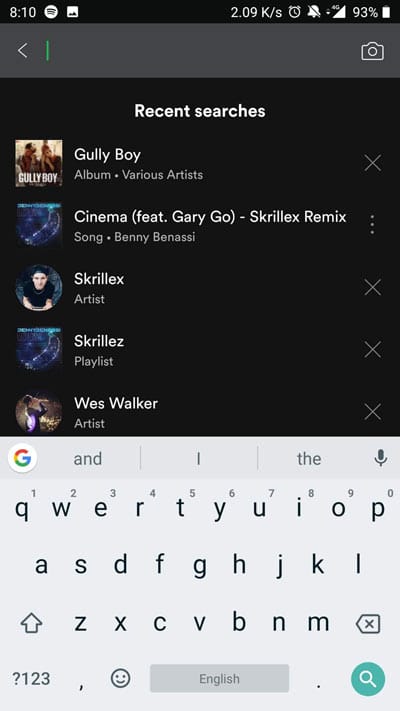**Detailed Caption:**

This image is a screenshot of a phone displaying a music application in dark mode, captured at 8:10 AM. At the top status bar, various icons are visible including a network signal symbol, an icon indicating 2.09K/s data usage, a stopwatch symbol, a muted bell icon, a 4G network symbol, and a battery level at 93%.

Below the status bar, there is a gray banner with a white left arrow (indicating a previous page or back option), a straight green line, and a camera icon on the left side. The main content under the gray banner falls under the "Recent Searches" section, showcasing multiple thumbnails and corresponding text.

The first thumbnail, labeled "Gully Boy," displays an image of two people, although the image is unclear, making it difficult to identify their genders. Adjacent to this thumbnail, the text "Gully Boy" appears in white, followed by "Album • Various Artists" and a gray 'X' icon on the left side, likely for deleting the search entry.

The next entry features a thumbnail with an ocean scene and some green writing. The accompanying text reads "Cinema feat Gary Go - Skrillex Remix by Benny Benassi." Below this, a thumbnail of an individual is displayed with the name "Skrillex" labeled as the artist. Another thumbnail showing an ocean image with green lettering indicates a "Skrillex Playlist."

Further down, there is a thumbnail of a person labeled "Wes Walker." 

Occupying the bottom third of the screen is a QWERTY keyboard, incorporating the Google symbol in the upper-left corner, a green circle containing a microscope symbol, and the standard keyboard lettering.